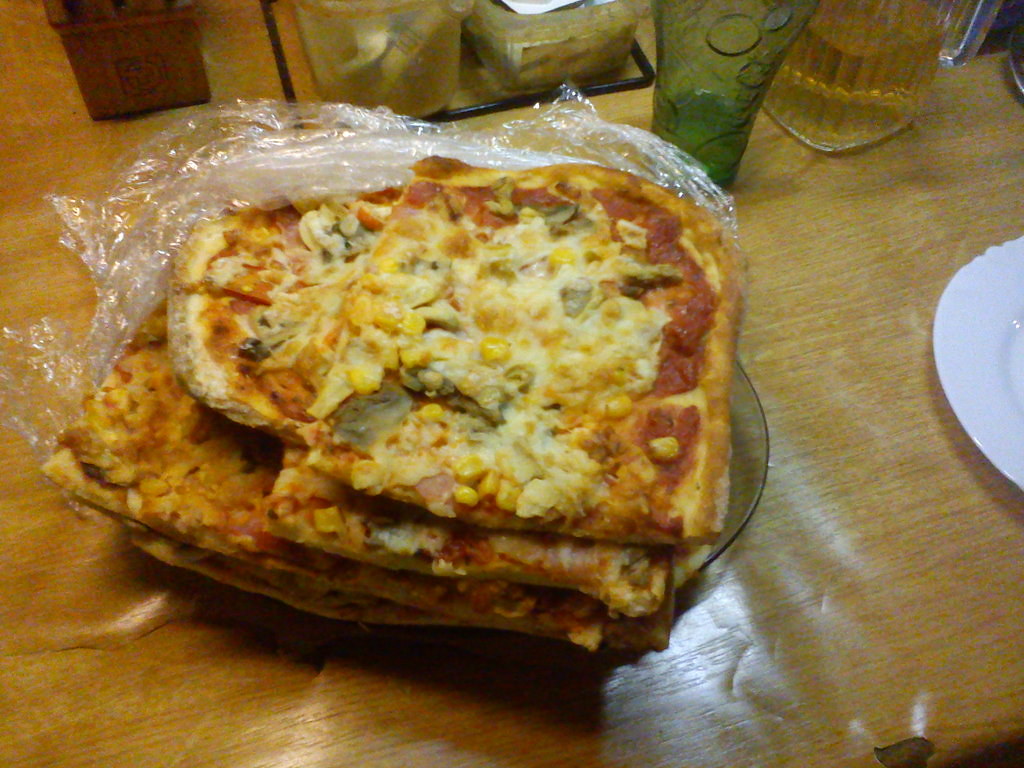On a light brown wooden tabletop, a stack of cold, square-cut pizza sits unappetizingly on a partially visible clear glass plate, with torn plastic wrap around it. The pizza appears old and sloppy, with toppings including green vegetable matter, sweet corn, olives, and some other pieces that might be ham. The crust is a golden brown color, and some of the sauce is visible in clumps. To the right of the pizza is a white plate, and in the background on the right are some glass cups and containers. The scene looks messy and somewhat uninviting.